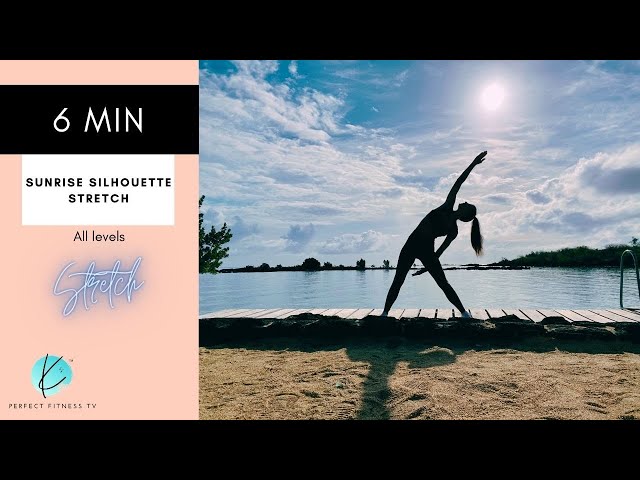The image showcases an advertisement for a 6-minute "Sunrise Silhouette Stretch" program, intended for all fitness levels, and available on Perfect Fitness TV. The ad features a striking silhouette of a woman performing a yoga pose on a wooden boardwalk by the edge of a lake, with a backdrop of brown sand and gentle clouds in a brilliantly blue sky. The woman, sporting a ponytail, has her body bent backward, with one arm extended upwards seemingly touching the sun, and the other arm extending downward. Her legs form an upside-down V shape. The text on the left side of the image includes the program's title in a combination of white and black font over a peach pink graphic background, with a blue circle housing the letter "K" or a yoga pose icon above "Perfect Fitness TV." The ad is bordered by thick black bars on the top and bottom, framing the serene and invigorating scene designed to inspire viewers to engage in this accessible and quick stretch routine.